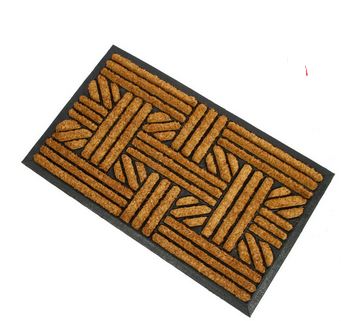This is a photograph of a heavy-duty doormat with a grayish-black rubber trim. The mat itself features a black and brown color scheme with intricate patterns made of bristly fibers. The design consists of three sets of horizontal and vertical brown bars which intersect to form a cross-like pattern across the mat. Additionally, there are lines running diagonally across the crisscrossed bars, altogether making nine horizontal lines, twelve vertical lines, and twenty-four diagonal lines. The mat is oriented diagonally in the photo, highlighting its detailed and structured pattern.